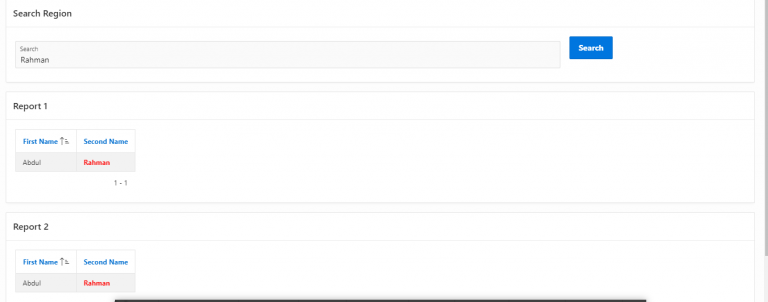The screenshot captures a computer interface within a certain application, displaying a predominantly white background. At the top of the screen is a horizontal search bar. In this search bar, the user has typed "RAHMAN," with a blue search button positioned to its right.

Beneath this search bar lies a white rectangular section labeled "Report One." This section details the first name "Abdul" and the second name "Rahman," accompanied by a label reading "1:1" just below the names.

A second report, labeled "Report Two," is located below the first report. This report contains the same first name "Abdul" and the second name "Rahman," but distinguishingly, the second name is highlighted in bright red, unlike the black text of the first report. The bright red matches the text in the search bar, possibly indicating a search result or query related to an area search for an individual named Rahman.